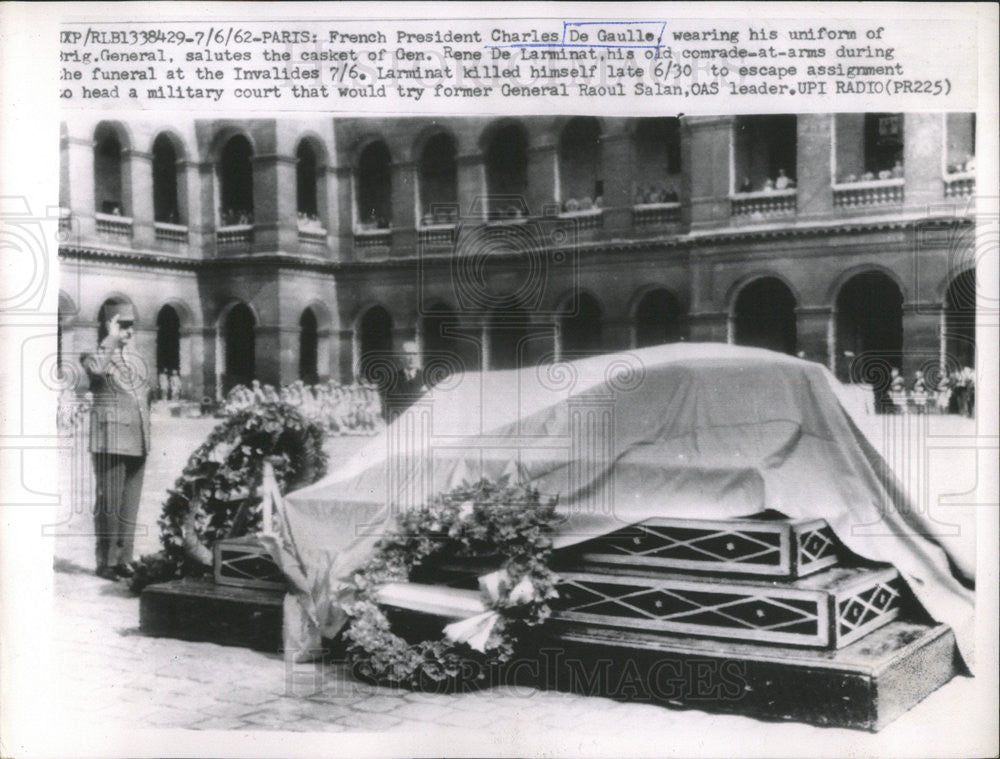This vintage black-and-white photograph, likely a newspaper clipping dated July 6, 1962, captures a solemn scene during the funeral of General René de Laramont at the Invalides in Paris. The central focus is a casket, draped with a sheet and adorned with large wreaths on a three-tiered platform, set on a brick roadway. To the left, French President Charles de Gaulle, clad in his Brigadier General's uniform, solemnly salutes his late comrade-in-arms. In the background, a grand two-story building with cathedral-like arches on both levels is visible, with people standing on the balconies and in the porticos, observing the ceremony. The photograph's title reads, "7-6-62 Paris, French President Charles de Gaulle, wearing his uniform of Brigadier General, salutes the casket of General René de Laramont, his old comrade-at-arms, during the funeral at the Invalides." The text also notes that General Laramont took his own life on June 30 to avoid leading a military court against former General Raoul Salan.